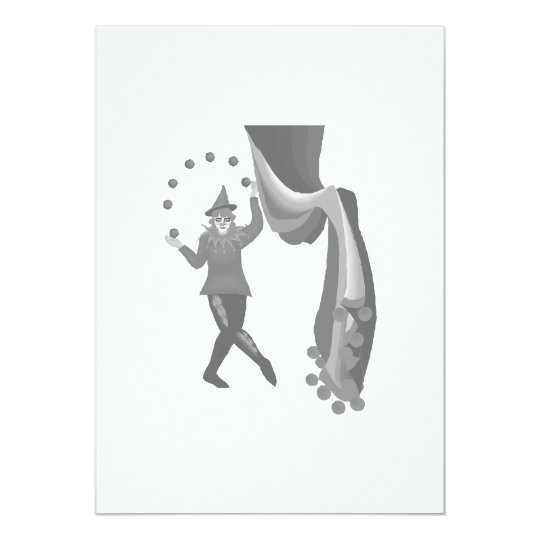This is a vertically aligned, rectangular image with a solid light gray background, bordered by a thicker gray margin on the right side and bottom, giving it the appearance of a card. Centered in the image is a graphic illustration of a Joker engaged in a juggling act. The Joker is adorned in a traditional outfit consisting of a pointed hat, a long-sleeved, dark gray top with a collar, and pants with decorative patterns down one leg. The Joker is shown juggling an arc of seven small gray balls above its head. 

To the right of the Joker, a tall, dark gray scarf with round circles at its base extends upwards, ending at the same level as the Joker's feet on the card. A curtain-drawn background frames the Joker, suggesting a performance setting. The curtain has varying shades of gray and white and appears to be opened to reveal the Joker, emphasizing the theatrical theme of the illustration. The entire scene, rendered in detailed shades of gray, depicts the animated essence of a digital graphic creation, representing a playful and entertaining spectacle.